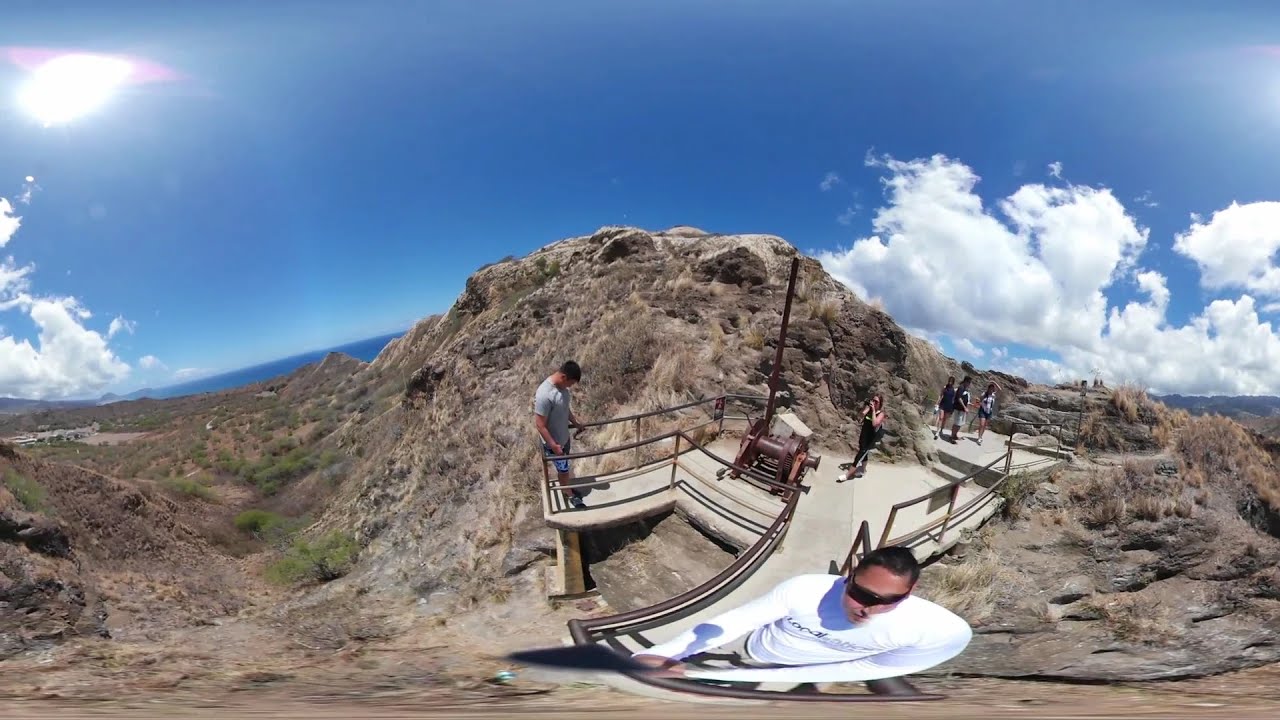The image showcases a wide-angle, 360-degree view taken during the daytime from a high vantage point in a hiking area. Central to the scene is a man, likely holding a camera on a selfie stick, who appears to be in the foreground. He has short black hair, wears dark sunglasses, and a tight, long-sleeved white shirt with black lettering across the chest. This man stands on the edge of a light gray concrete walkway, which is flanked by a railing made of brown metal bars. 

On the left side of the walkway, another man in a gray shirt and blue shorts stands against the barrier, looking down at his phone. Behind these two figures, the walkway curves along a rocky mountain formation, which arches with varying shades of gray and some patches of greenery. In the background, farther along the path, three individuals can be seen walking. On the right side, a woman in a black jumpsuit stands facing a seated man, holding a camera.

To the far left, there’s a small valley lush with green vegetation and spotted with patches of dirt. Above the scene, white and gray clouds partially fill the sky, with a vivid blue expanse beyond them. The upper left corner of the image is particularly bright, with a white sun encircled by a hint of purple. The entire setting exudes an atmosphere of being outdoors in nature, amidst the rugged beauty of a mountainous landscape.